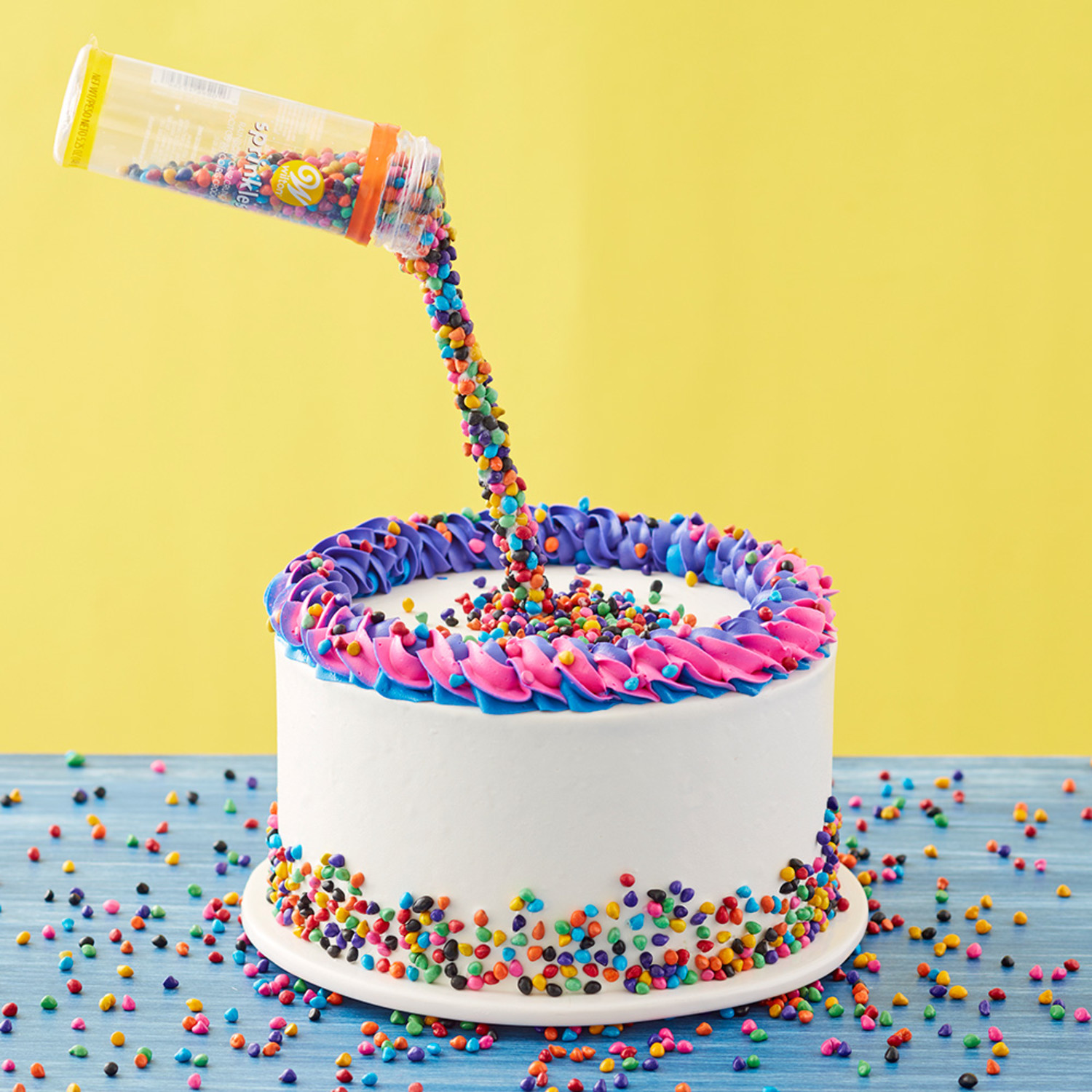This professional photo captures a vividly decorated one-tier cake, reminiscent of a feature in a high-end baking magazine. The cake is enveloped in smooth white frosting, adorned with a wavy fringe of blue, pink, and purple icing along the top edge. It sits on a white plate, which rests on a visually appealing blue wooden table, complementing the cake’s vibrant theme. The table is scattered with assorted sprinkles in an array of colors, including blue, red, yellow, purple, green, pink, and darker hues like black or brown, adding to the festive atmosphere.

The cake's base is bordered by a dense layer of these multicolored sprinkles, creating a playful and eye-catching contrast against the white frosting. The top of the cake features a dynamic display where a stream of sprinkles appears to be magically pouring from a suspended sprinkle jar, as if an invisible hand is artfully decorating the cake. This creative flourish is enhanced by more sprinkles piled up in the center of the cake, partially surrounded by the colorful fringe.

Behind the cake, a cheerful yellow wall adds a warm and inviting backdrop, making the overall presentation even more delightful. The meticulous arrangement and vibrant colors make the cake look not only delicious but also visually stunning, capturing a sense of fun and celebration.